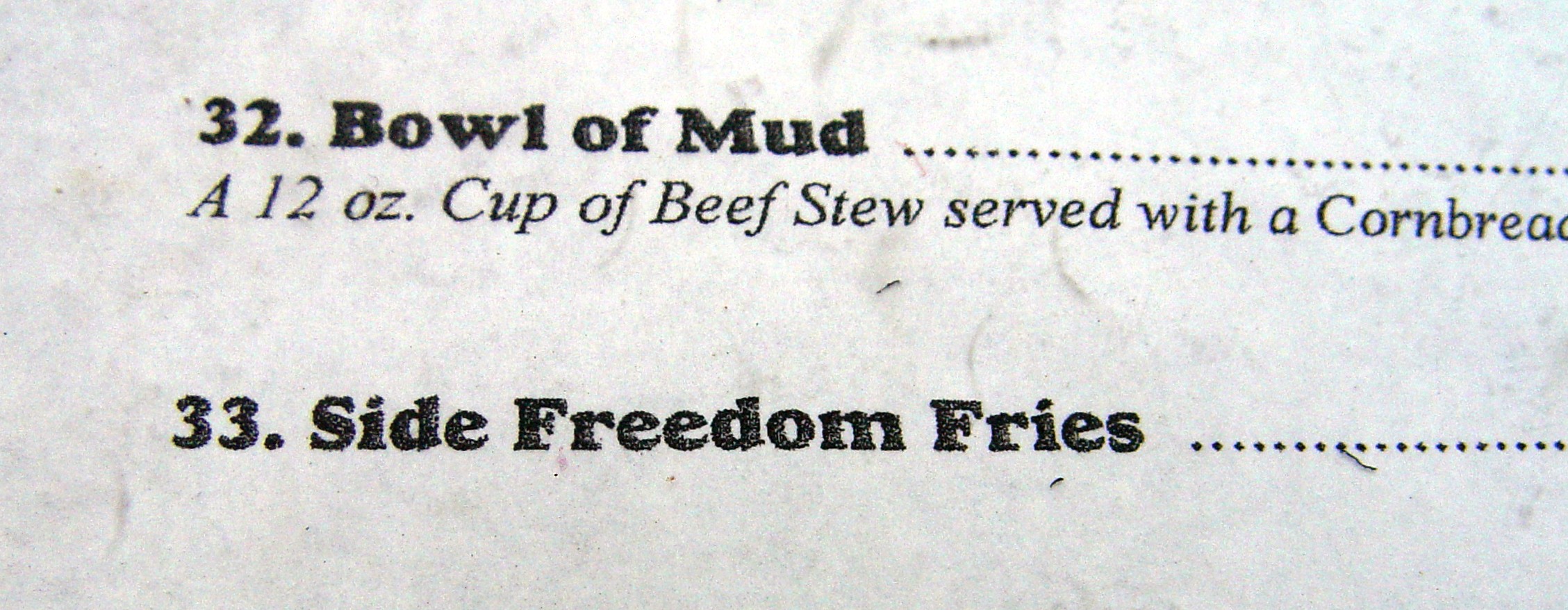This detailed, zoomed-in black-and-white image captures a segment of a vintage menu. The photograph, presented in a horizontally-oriented landscape format, prominently features two menu items. Boldly listed at the top is "32. Bowl of Mud," followed by dotted lines leading to the right edge of the frame where the price would typically be displayed, though it is cut off in this image. Below this, in a thinner and unbolded font, the menu describes this item as "a 12-ounce cup of beef stew served with cornbread," with the remaining text truncated by the photo's edge.

Beneath this entry, the number "33." is also bolded, accompanied by the words "Side Freedom Fries" in a similarly bold font. This line is followed by another series of dots extending toward the right, again cutting off before reaching the price. The entire image is characterized by a grainy texture, indicative of a scanned reproduction of the original document, with various black streaks and speckles scattered across the white background, adding to its vintage feel.